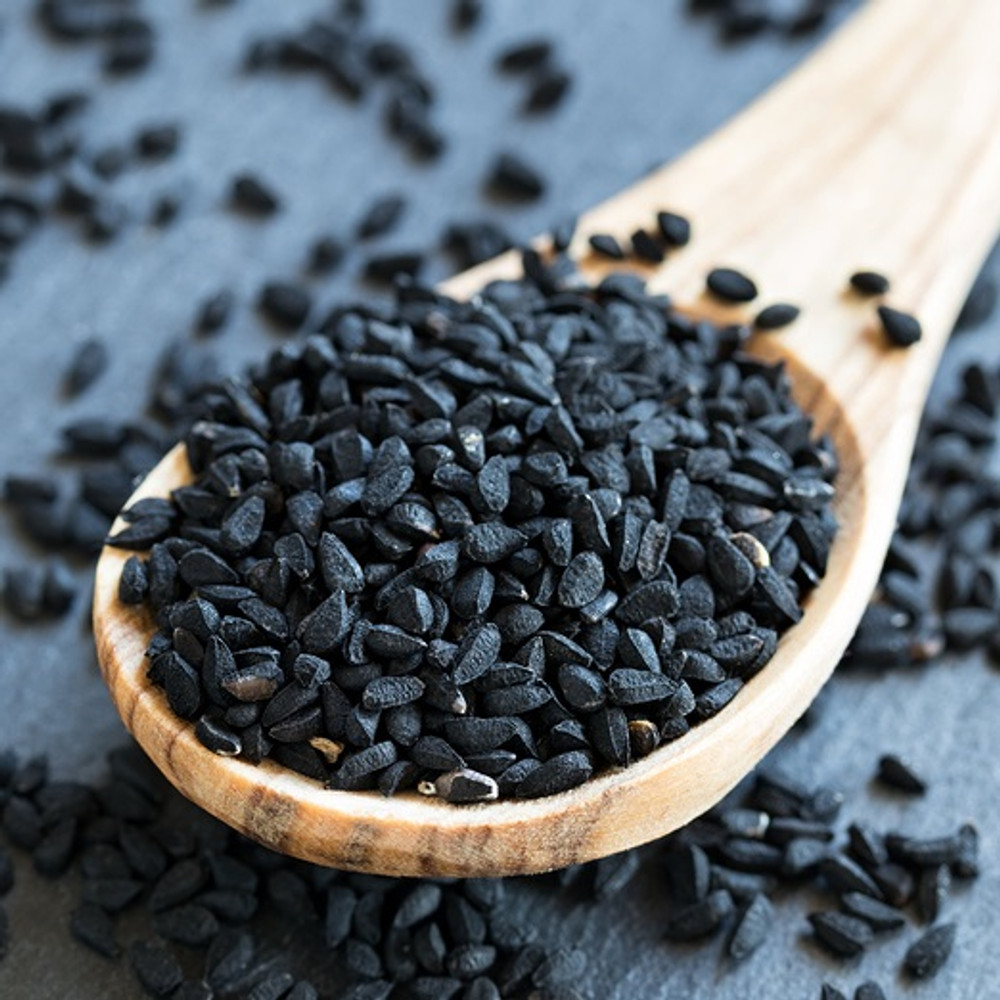The photograph is a close-up of a rustic wooden spoon, light beige in color, filled with numerous small black seeds resembling tiny slices of oranges or pieces of coal. The spoon, brimming with these seeds, is artistically laid out over a grey wooden surface, which is also scattered with additional seeds, enhancing the visual impact. While the spoon extends out of the upper right-hand corner of the frame, only the foreground elements, particularly the spoon and the seeds inside it, are in sharp focus. The background seeds and surface remain blurred, drawing attention primarily to the heaping spoonful of seeds, suggesting their culinary use pending further preparation.